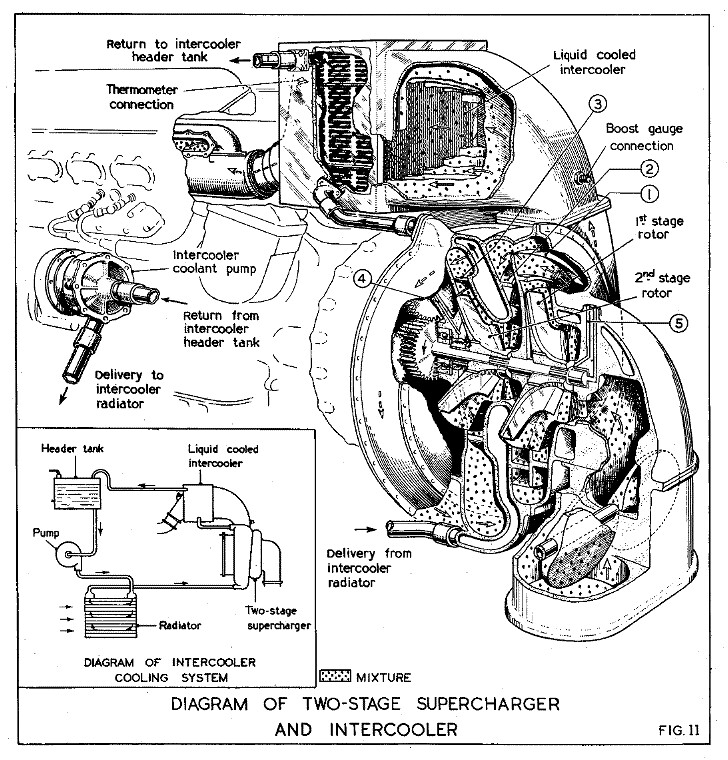This black and white image is a detailed diagram of a two-stage supercharger and intercooler, labeled as "Figure 11." The caption at the bottom center reads "diagram of two-stage supercharger and intercooler" in black text against an all-white background. The majority of the image features a cross-sectional view of the supercharger and intercooler, labeled with parts such as liquid-cooled intercooler, first and second stage rotors, return to intercooler header tank, thermometer connection, intercooler coolant pump, return from intercooler header tank, delivery to intercooler radiator, and boost gauge connection. These components are intricately connected with tubing, pipes, and various engine parts, with arrows indicating the flow of the liquid.

On the bottom left, there's a rectangular inset labeled "diagram of intercooler cooling system," showing an outlined, simplified version of the main diagram. This section depicts the header tank, liquid-cooled intercooler, two-stage supercharger, radiator, and pump, with arrows indicating the direction of flow. This highly detailed illustration provides a comprehensive view of the inner workings and connections within the two-stage supercharger and intercooler system. 

Overall, this manual-like image offers an in-depth look at the equipment, combining detailed cross-sectional views with simplified flowcharts for clarity.